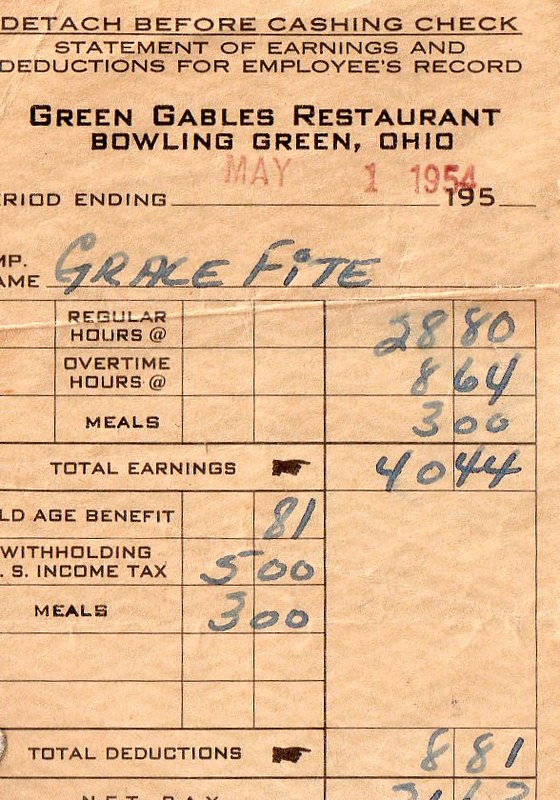The image displays an aged, weathered pay stub from Green Gables Restaurant in Bowling Green, Ohio, dated May 1, 1954. The slightly folded, grainy paper, which is an off-white with a brownish hue, features the text predominantly in black font. At the top, it reads in all caps: "DETACHED BEFORE CASHING CHECK, STATEMENT OF EARNINGS AND DEDUCTIONS, FOR EMPLOYEE'S RECORD." Below that, in darker text, it states the restaurant's name and location, followed by "PERIOD ENDING MAY 1ST, 1954." The employee's name is Grace Fite. Her regular hours amount to $28.80, with additional overtime hours recorded as $8.64, and meals at $3.00, making her total earnings $4044. The deductions listed include an age benefit of $81, income tax of $500, and meals at $3.00, bringing total deductions to $881.